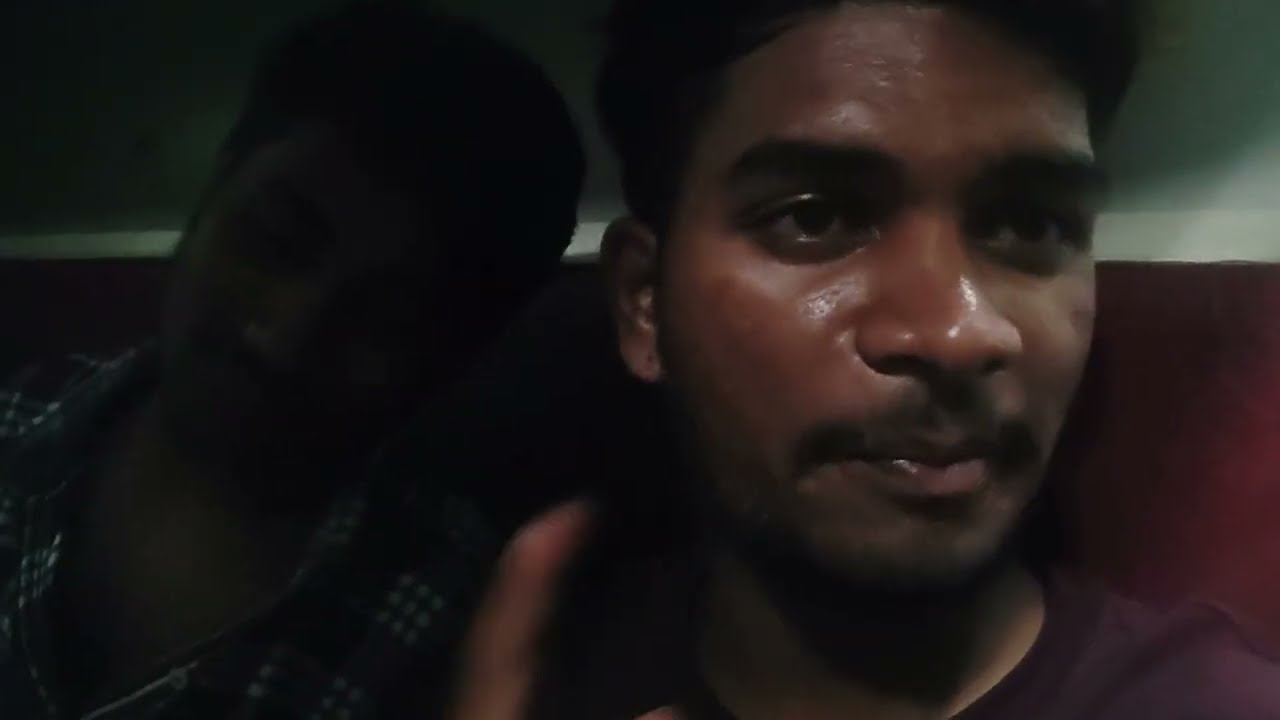This photograph features an up-close shot of two young men, possibly of Indian or Middle Eastern descent, with slightly dark brown skin and short black hair. The man on the right is bathed in sufficient light and is wearing a maroon-colored t-shirt. He looks somewhat tired, with a thin black mustache and lips slightly pursed, gazing intently toward the right side of the frame. His forehead is partially cropped out due to the photo's composition. 

To his left stands another man, largely cast in shadow, making him less discernible. He too has black hair and a mustache, but his facial expression is obscured by the poor lighting. He is dressed in a plaid button-down shirt with the top few buttons undone. He appears to either have his eyes closed or be looking downward, with his head slightly tilted towards his companion.

The background of the image transitions from white and gray at the top to red at the bottom, contributing to the slightly blurry ambiance of the photograph.